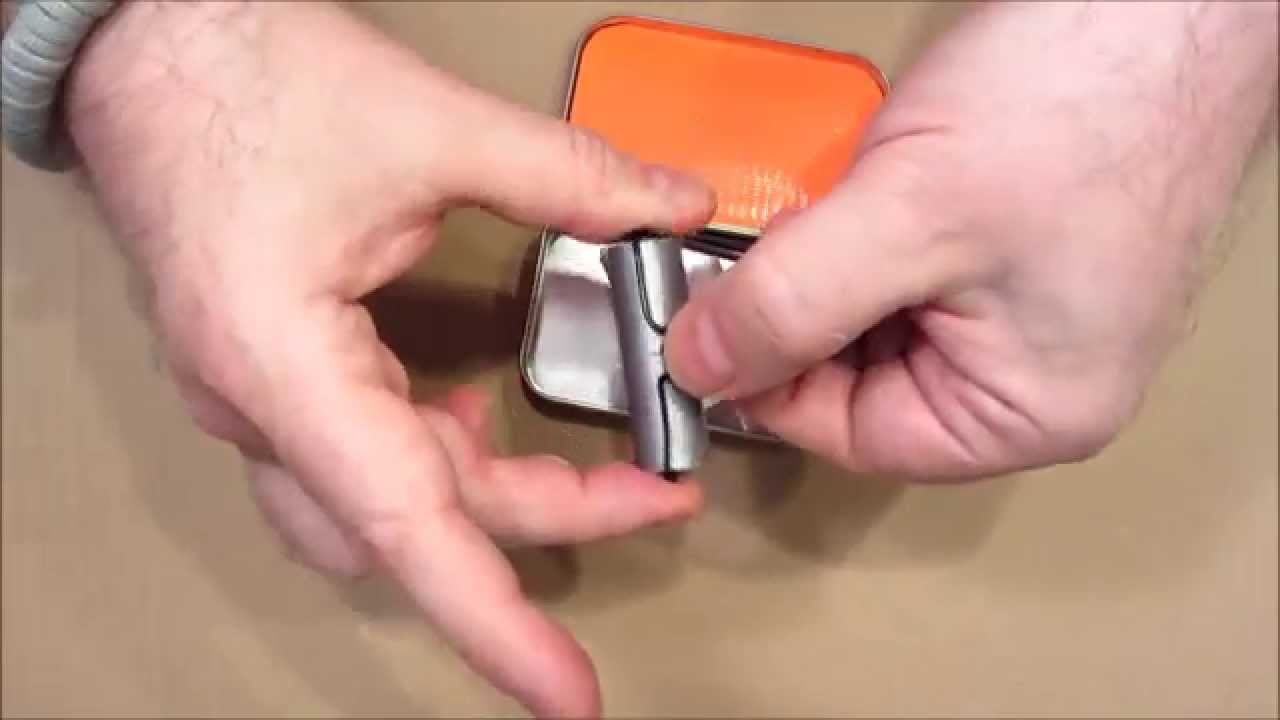This is a color photograph depicting a pair of pale, somewhat hairy male hands. These hands are engaged in demonstrating how to open a silvery grey latch or buckle, which is being held between the middle finger and thumb of one hand while being pinched by the other. The individual appears to be of Caucasian ethnicity. In the background, there's a rectangular tin that resembles a mint tin with an orange and white interior, indicating that the tin is open. On the right wrist, a bracelet or watch band is faintly visible. The beige background contrasts the objects in focus. The image is slightly blurry, adding a touch of ambiguity to the exact nature of the metallic object being handled.